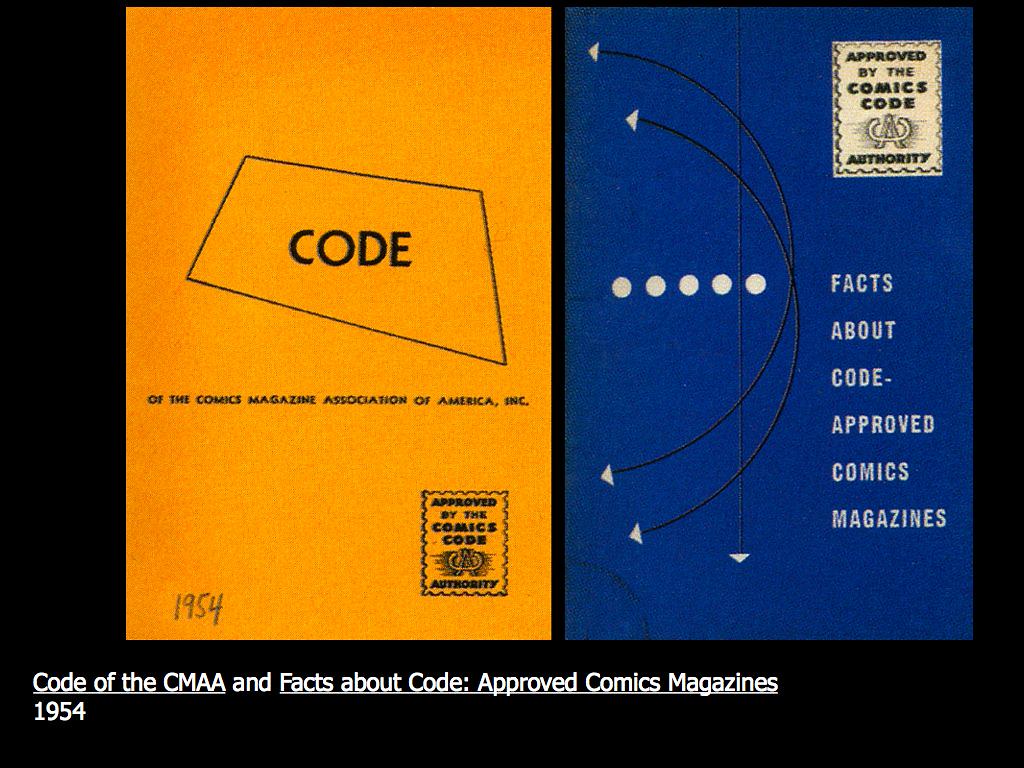The image showcases two pages, appearing to be scans, each representing distinct sections related to the Comics Code Authority from 1954. On the left side, there is a mustard yellow page featuring the text "Code of the Comics Magazine Association of America" in black, accompanied by a handwritten "1954" in the bottom left corner. At the bottom right, it is stamped "Approved by the Comics Code Authority" along with their logo. The page on the right contrasts with a royal blue background. In the top right, it again reads "Approved by the Comics Code Authority" in black and white. The center of this blue page is decorated with five white horizontal dots, curved lines with arrows, and a downward-pointing arrow, with the text "Facts About Code Approved Comics Magazine" in white. Below these scans, in small white text, it is noted, "Code of the CMAA and Facts About Code Approved Comics Magazines 1954."